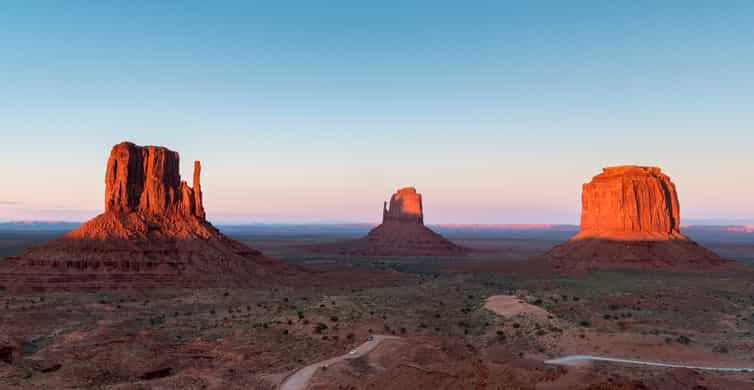The image captures a striking desert landscape dominated by three towering buttes or mesas, reminiscent of the southwestern United States. These reddish rock formations are spread evenly across the arid terrain, each distinct yet harmoniously part of the scene. The leftmost butte, slightly slanted at the base, reflects the sun's rays, glowing brightly. The central butte, set further back, casts dramatic shadows, emphasizing its rugged texture. The rightmost formation appears rounder and is bathed in sunlight, showcasing a vibrant red hue. The landscape below is sparsely vegetated with patches of grass and resilient shrubs dotting the barren ground. The sky above transitions smoothly from a whitish hue near the horizon to a deeper sky blue as it ascends, completing this picturesque desert vista.